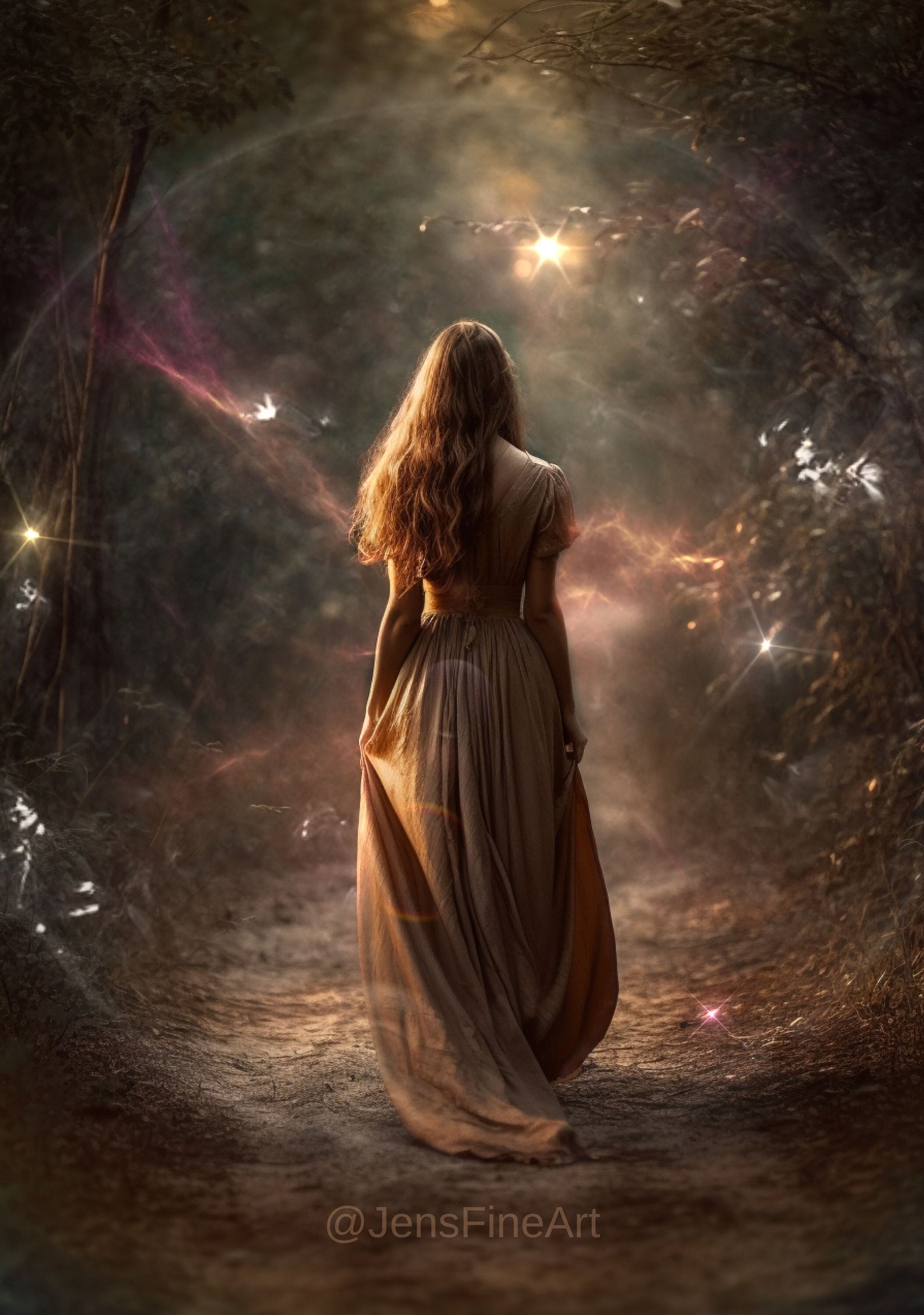The image captures a woman from behind as she walks down a fantasy-themed pathway adorned with glowy lights. Her long blonde hair cascades down to her midsection, and she wears a tan-colored dress. She holds the sides of her dress with both hands. The pathway beneath her feet is composed of dirt and sand, adding a rustic element to the fantastical setting. The texture of the picture has some areas that are a bit blurry, contributing to the dream-like quality of the scene. At the bottom of the image, a light-text watermark reads "At Jen's Fine Art."